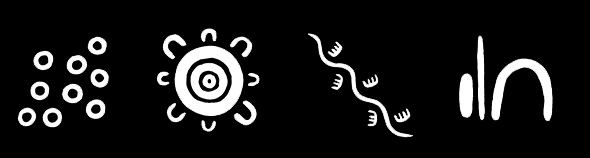This black and white image features four distinct illustrations arranged side-by-side against a black background. The first illustration consists of nine white, unshaded rings, arranged haphazardly yet forming three rows of three. The third row is positioned slightly higher than the first two. The second illustration resembles an abstract sun or flower with concentric circles at its center. These consist of alternating white and black rings, surrounded by U-shaped rays or petals. The third illustration displays a squiggly diagonal line with shapes resembling four-clawed footprints, evenly spaced and aligned along its ridges, suggestive of a tail-dragging motion. Lastly, the fourth illustration features an upside-down U shape adjacent to two vertical lines of differing height: one tall and slender and the other short and broad. The overall composition of the artwork is more landscape-oriented than portrait.